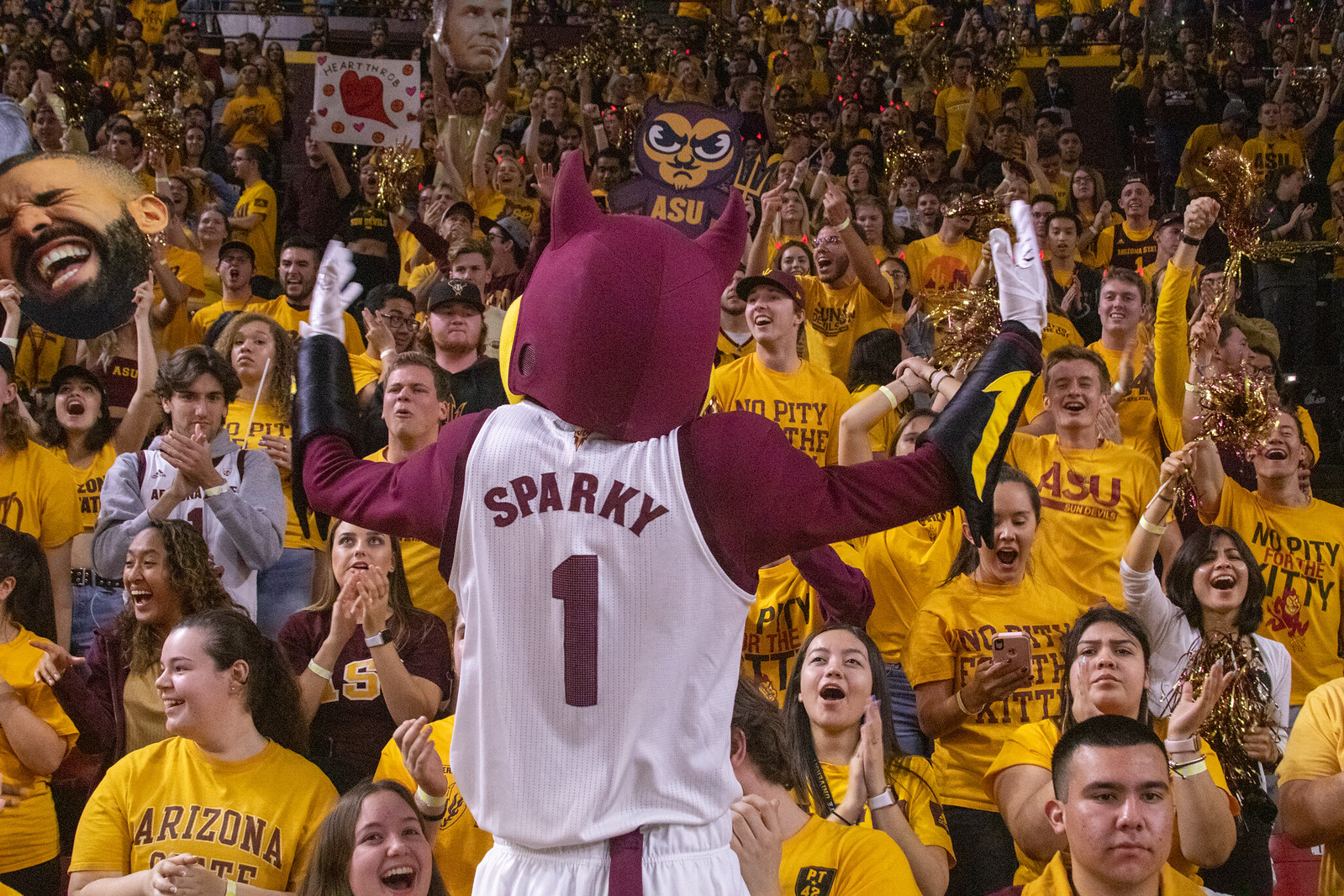In this vibrant, full-color photograph taken at a lively Arizona State University sports event, an enthusiastic crowd of college students fills the stadium, predominantly wearing yellow T-shirts emblazoned with "ASU" or "Arizona State" in red. The thrill and excitement are palpable as the attendees cheer, clap, and smile, many waving gold tassels. Central to the image is the iconic ASU mascot, Sparky, facing the crowd. Sparky, a red devil-like figure, dons a white uniform with the name "Sparky" and the number one in red. He sports a distinctive red hat, red arms, white gloves, and black gauntlets with yellow trim. Among the sea of exuberant fans, several hold up large, eye-catching signs, including giant head cutouts of comedian Will Ferrell and singer Drake, an ASU Devils mascot sign, and a white sign adorned with hearts. The photograph, rectangular in shape and likely taken indoors, captures a moment of shared elation and school spirit among the young audience members.